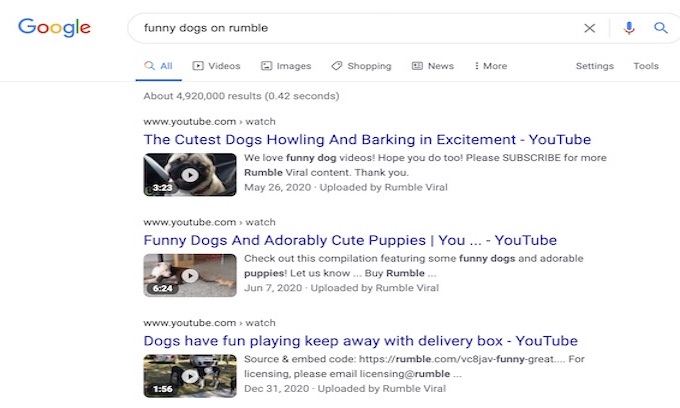The image displays a Google search results page for the query "funny dogs on Rumble." The search results are sorted under various categories including "All," "Videos," "Images," "Shopping," "News," "More," "Settings," and "Tools." From the provided search query, three notable video results, all hosted on YouTube and uploaded by Rumble Viral, are visible:

1. **Cutest Dogs Howling and Barking in Excitement**   
   - **Date:** May 2020  
   - **Video Length:** 3 minutes and 23 seconds  
   - **Description:** This video features an assortment of the cutest dogs, howling and barking in sheer excitement.

2. **Funny Dogs and Adorably Cute Puppies**  
   - **Date:** June 2020  
   - **Video Length:** 6 minutes and 24 seconds  
   - **Description:** A delightful compilation of funny dogs and irresistibly cute puppies.

3. **Dogs Have Fun Playing Keep Away with Delivery Box**  
   - **Date:** December 31, 2020  
   - **Video Length:** 1 minute and 56 seconds  
   - **Description:** Watch as these playful dogs enjoy a game of keep away using a delivery box.

All three videos showcase endearing moments of dogs and puppies.